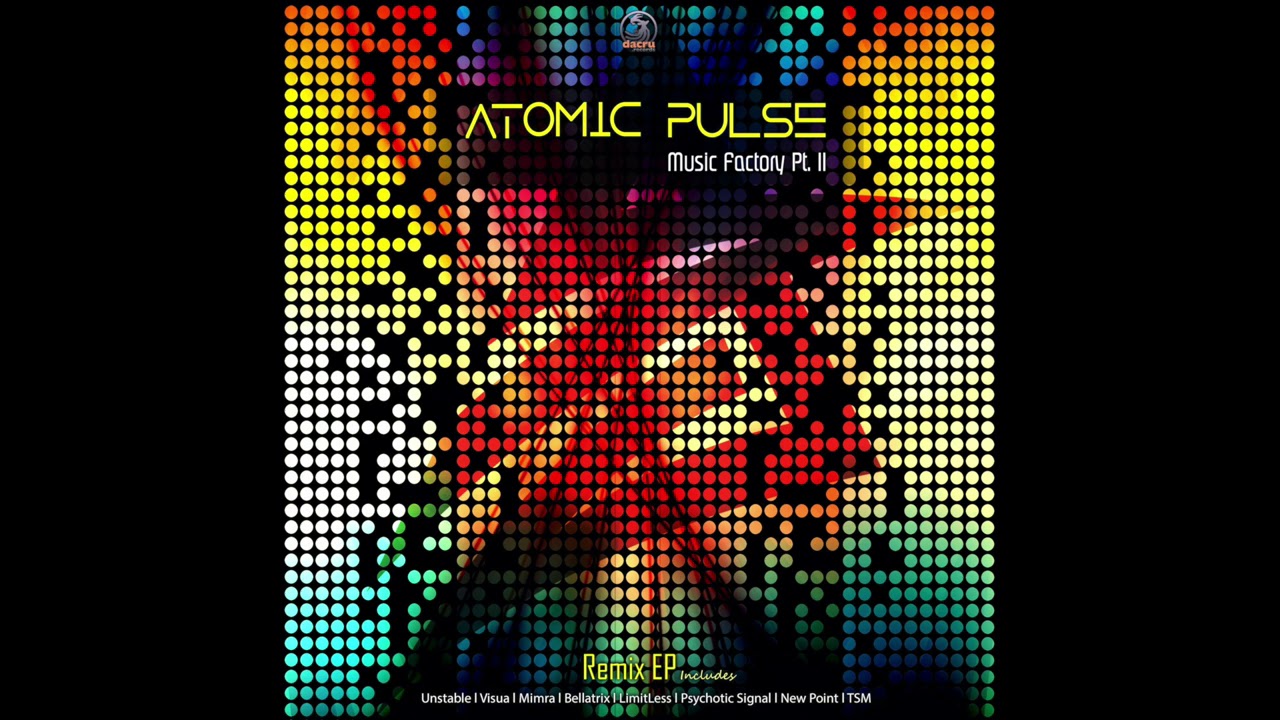This vibrant album cover features a striking array of small, multicolored circular dots arranged in numerous rows and columns. Set against a pure black background on both sides, the dots transition from warm hues of orange and yellow at the top to deeper blues and greens towards the bottom, reminiscent of a rainbow gradient. In the center, illuminated in bold yellow lettering, is the title "Atomic Pulse," with "Music Factory Part 2" appearing just below it in smaller white letters. Below this central title, an abstract, geometric figure resembling a stylized 'Z' with an additional line can be observed. The bottom of the cover lists more text, starting with "Remix EP" in yellow, followed by "Includes" and a series of track names in smaller white text: Unstable, Visual, Memera, Bellatrix, Limitless, Psychotic, Signal, Newpoint, and TSN. The overall composition and vibrant color scheme give the impression of a digital art piece or a nostalgic reference to a lit-up, multi-colored pegboard toy.